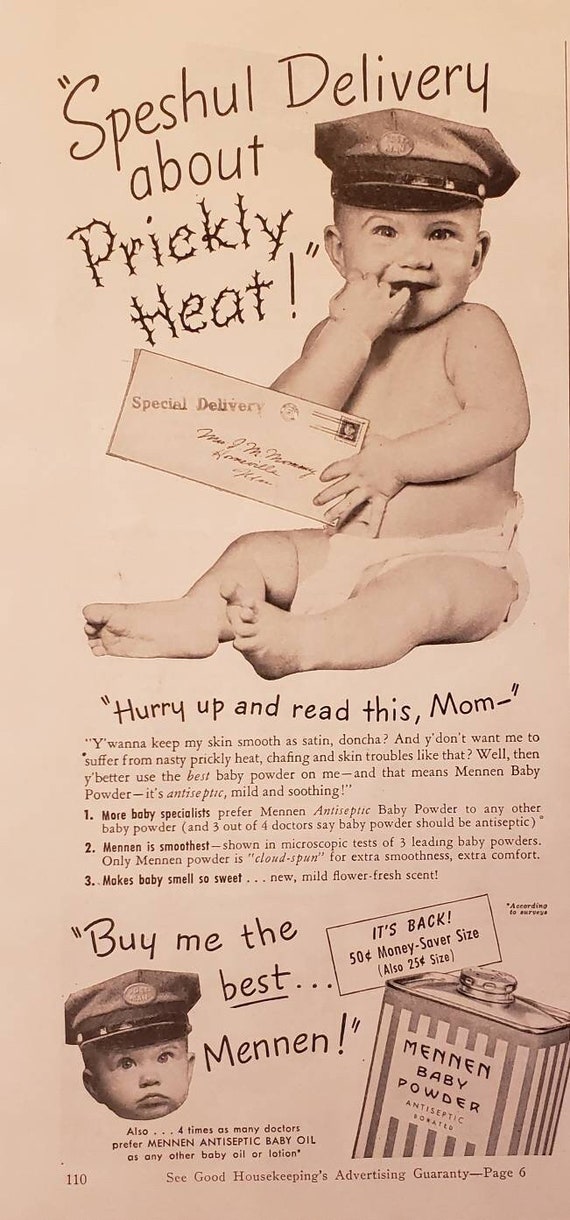The image is a page from an old magazine, featuring a vintage advertisement for Menin Antiseptic Baby Powder. The background has a light brown, sepia-toned color, giving it an aged appearance. At the top of the page, the headline in quotes reads, "Special Delivery about Prickly Heat," with "prickly heat" styled in a thorny font. Below this headline, a large picture depicts a joyful baby wearing only a diaper and a postman's hat, holding an envelope marked "Special Delivery" and smiling directly at the camera.

Beneath the image, the text addresses parents, urging: "Hurry up and read this, mom. You want to keep my skin smooth and satin, don't you? And you don't want me to suffer from nasty prickly heat, chafing, and skin troubles like that. Well, then you better use the best baby powder on me, and that means Menin Baby Powder. It's antiseptic, mild, and soothing." The ad goes on to claim that "More baby specialists prefer Menin Antiseptic Baby Powder to any other baby powder. And three out of four doctors say baby powder should be antiseptic. Menin is the smoothest, shown in microscopic tests of three leading baby powders. Only Menin Baby Powder is close-spun for extra smoothness and extra comfort, making baby smell so sweet with a new mild flower fresh scent."

Further down, another image shows a close-up of the same baby wearing the cap, accompanied by the tagline "Buy me the best... Menin!" Next to this is an advertisement for Menin Baby Powder's packaging, illustrating cans labeled "Menin Baby Powder Antiseptic" with white striped designs, offering sizes in 50 cents (money saver size) and 25 cents. Beneath this, a footnote claims that "Four times as many doctors prefer Menin Antiseptic Baby Oil to any other baby oil or lotion," with a note referencing the "Good Housekeeping" advertising guarantee on page 110.